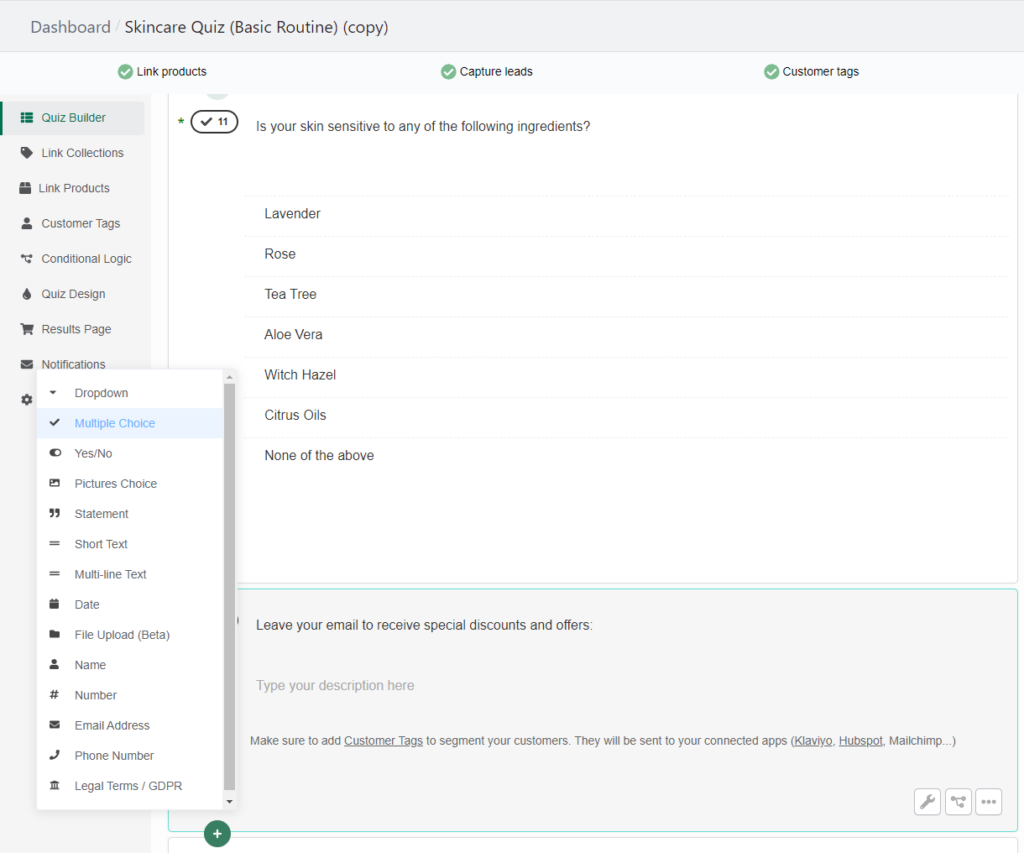### Descriptive Caption

This image showcases a detailed view of a skincare quiz dashboard within a software interface. At the top, the header reads: “Dashboard / Skincare Quiz Basic Routine Copy.” On the left sidebar, there is a vertical menu displaying various options, each accompanied by a representative icon. These options include:

- Quiz Builder (currently selected)
- Link Collections
- Link Products
- Customer Tags
- Conditional Logic
- Quiz Design Results
- Page Notifications
- Settings

Beneath the "Quiz Builder" section, a drop-down menu is visible, featuring multiple input types such as:

- Multiple Choice
- Yes/No
- Pictures Choice
- Statement
- Short Text
- Multi-line Text
- Date
- File Upload (Beta)
- Name
- Number
- Email
- Address
- Phone Number
- Legal Term/GDPR

Each item in this menu is also marked with a unique icon. On the right side of the interface, a preview of the quiz question is displayed. The quiz question, numbered 11, asks: “Is your skin sensitive to any of the following ingredients?” with options including Lavender, Rose, Tea Tree, Aloe Vera, Witch Hazel, Citrus Oils, and None of the Above.

Below this question, there is another prompt: “Leave your email to receive special discounts and offers,” followed by an input field with a placeholder text in a lighter font color: “Type your description here.” Additionally, there is a note to “Make sure to add customer tags to segment your customers,” with the phrase "customer tags" underlined and indicating integration with connected apps such as HubSpot, MailChimp, and Klaviyo.

At the very bottom, there are three function icons: a wrench, a share icon, and a more options icon (three dots).